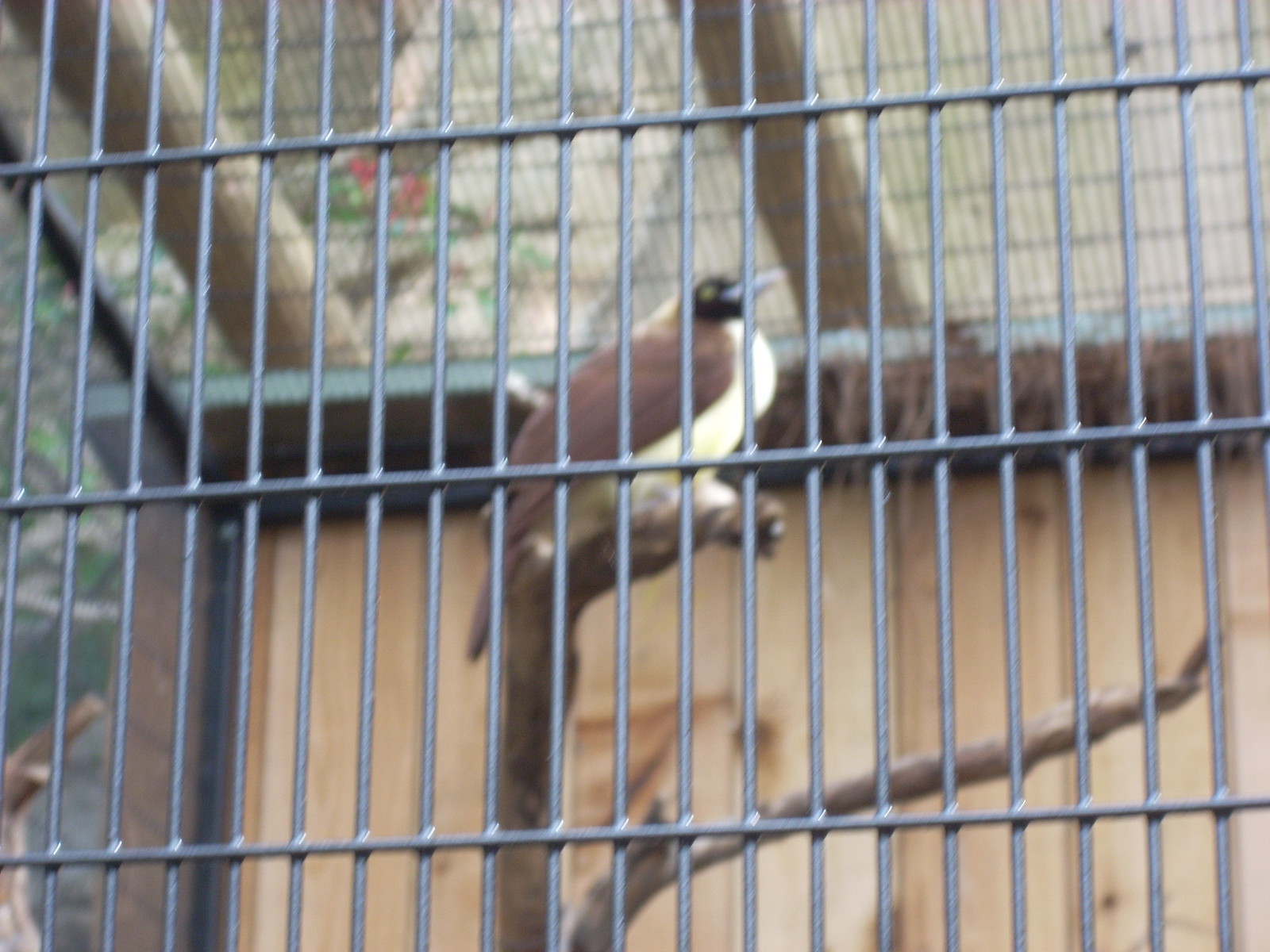This outdoor daytime photograph, rectangular at approximately six inches wide by four inches tall, captures an image of a bird inside a wire mesh cage, typical of a zoo enclosure. The cage features thick, fine black bars prominently displayed in the foreground, drawing immediate attention due to the camera's focus on them. These bars are horizontally aligned in three rows, with numerous thin vertical bars dividing the space. The top of the cage is covered in wire mesh, ensuring the bird remains contained while allowing it room to fly.

Beyond the cage's metal bars, though subtly blurry, the primary focus reveals a barren tree stump within the enclosure. Perched on one of the stump's branches sits a distinctive bird. This bird showcases a striking black head with a light green eye, transitioning to a long gray beak. Its chest and belly are white, contrasting with its predominantly brown wings and light brown back and tail feathers. The bird is facing right, its feet not visible from this angle.

The rear wall of the cage consists of a plain wooden background, likely oak, providing a rustic backdrop. The overall scene encapsulates the melancholy isolation of the bird within its structured yet naturalistic habitat.